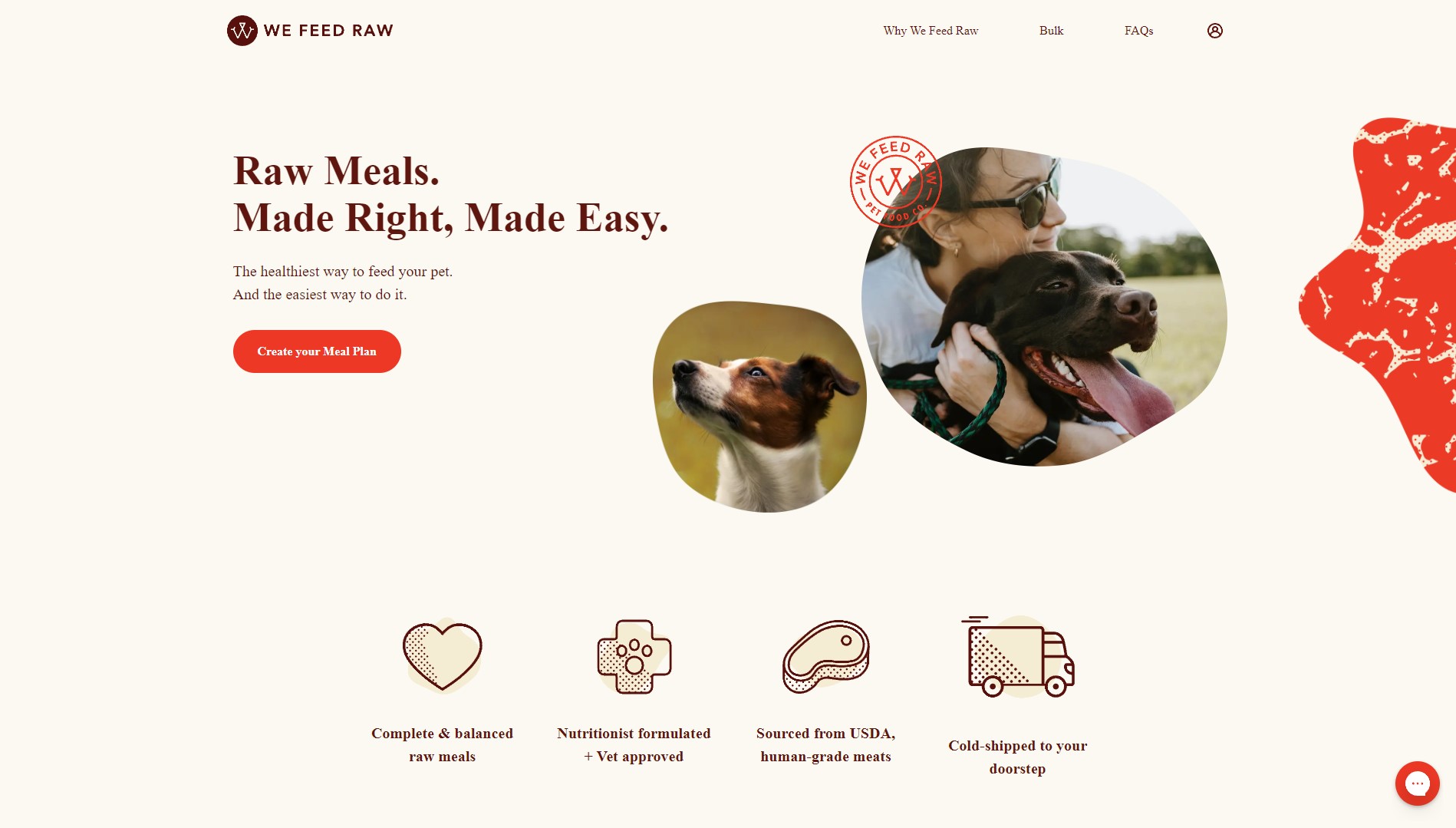The screenshot from a website features a light beige background at the top. On the left side, there's a black circular icon with a white 'W' inside it, next to the text "We Feed Raw" in black font. To the right of this are several drop-down menus or links labeled "Why We Feed Raw," "Bulk," and "FAQ." Additionally, there is an icon showing a human silhouette within a circle.

Beneath this top navigation bar, the text in black font reads: "Raw Meals, Made Right, Made Easy, The Healthiest Way to Feed Your Pet, and The Healthiest Way to Do It." Below this slogan is a prominent red button with white text that says "Create Your Meal Plan."

To the right of this text, there are two circular photos. The first, on the left, features a Jack Russell Terrier looking up and to the left, with a green background visible. The second, situated slightly above and to the right, shows a white woman embracing a black Labrador. Both are facing right, with the Labrador's mouth open and its pink tongue hanging out.